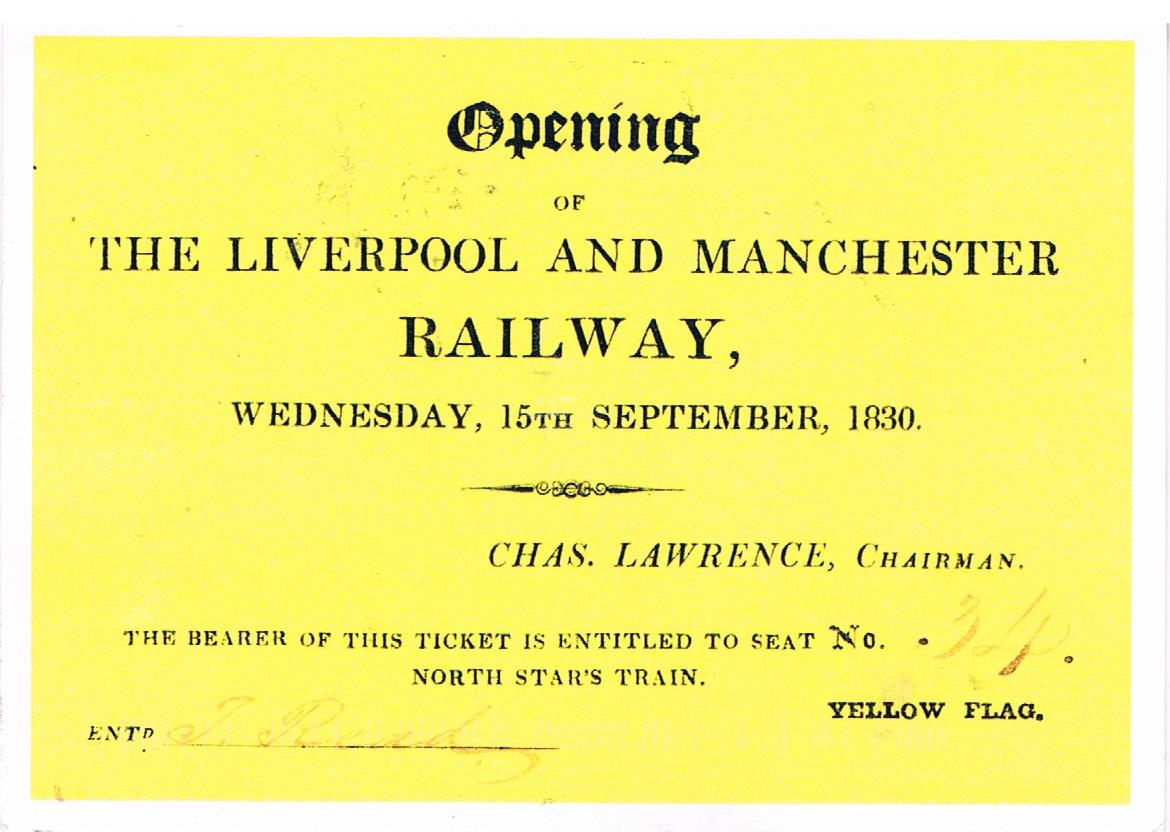This image features a bright yellow piece of paper, which appears to be a historical ticket. At the top of the ticket, in black text, it reads: "Opening of the Liverpool and Manchester Railway, Wednesday, 15th September, 1830. Chas (C-H-A-S) Lawrence, Chairman." Below this, there is a handwritten section in brown ink with a swirly font, indicating the number "34." Beneath the handwritten number, in black text again, it states: "North Stars Train." On the bottom left corner of the ticket, there are the letters "E-N-T" followed by a line, above which there is a signature. The bottom right corner of the ticket has the words "Yellow Flag" written in black text. The overall presentation of the ticket suggests it was an important document for attending the historic railway opening.